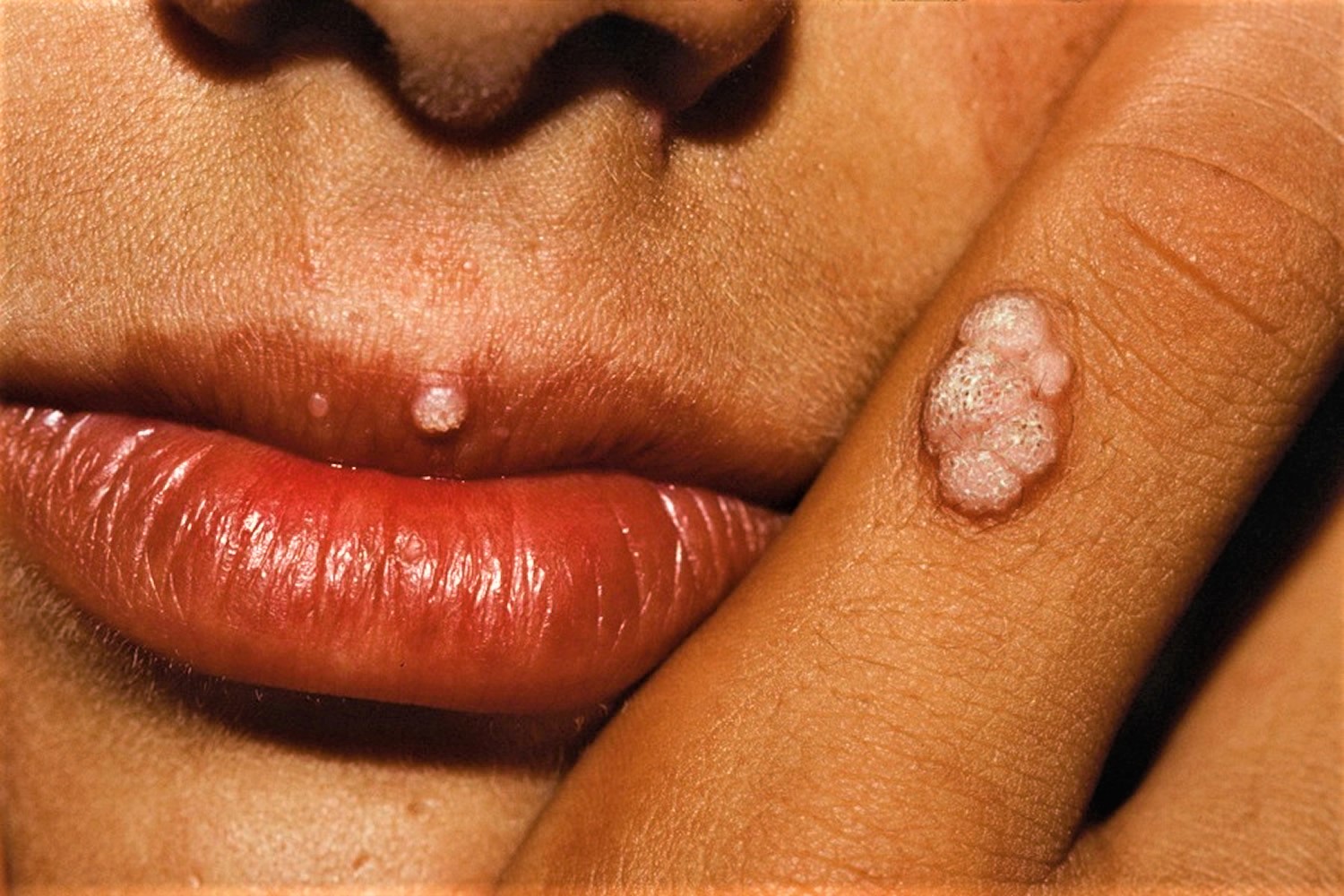This is a close-up photo likely of a woman, though the gender is somewhat ambiguous due to contrasting details. The focus is on her lips and the fingers she has raised to her mouth. Her skin is tan, and her lips are naturally red, appearing somewhat cracked, without lipstick. On her upper lip, there is a small white bump that looks like a sore, potentially filled with pus. Her finger, which is touching her lip, features a much larger white and red bump, resembling a boil or skin rash, with some brown specks. The sores on both her lip and finger suggest a skin condition or viral infection. The close framing of the image keeps the setting indistinct, highlighting only her lips and hand.